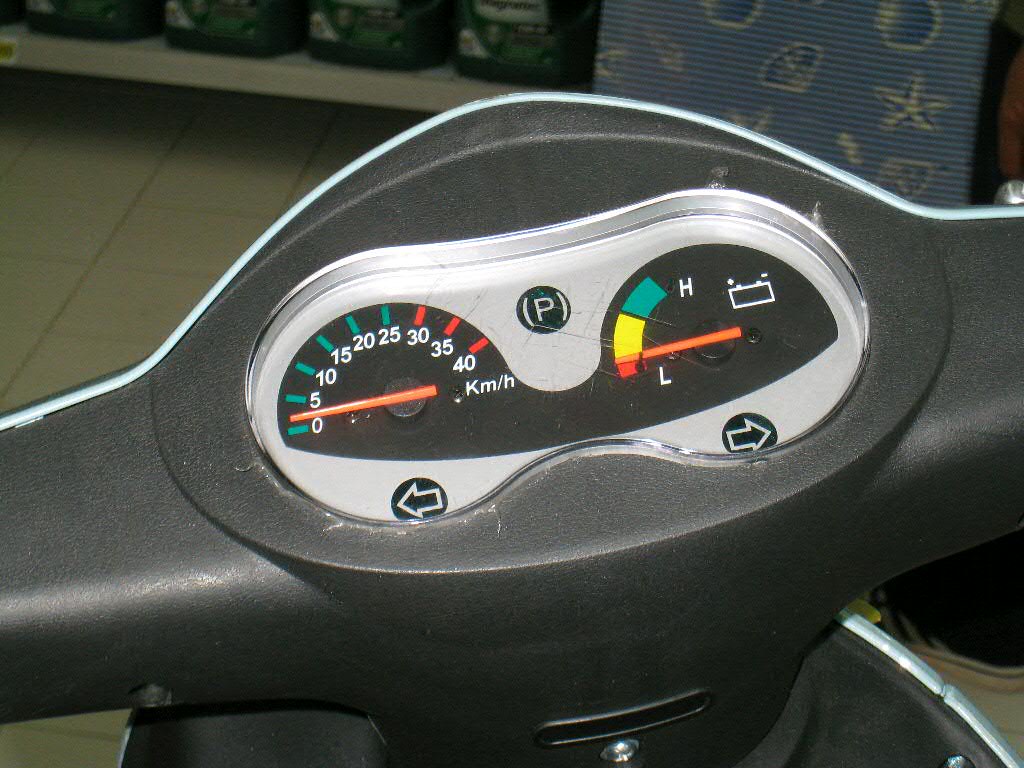This photograph captures the handlebar area of a mobility scooter, showcasing a variety of intricate details. At the center of the image is the scooter's display console, constructed from a dark gray, curved plastic handle with an oval opening in the middle. Although the full handlebars are cut off by the photograph's edge, a hint of their presence is visible.

The display's lower section features two directional arrows in white outlines on black circles: one pointing left and the other right. Prominently near the top of the display is another black circle inscribed with a capital letter "P" enclosed in parentheses, denoted in white text.

Two half-circle gauges dominate the dashboard, connected by a slender curving branch. Each gauge features an orange needle, both pointing to their lowest positions on the lower left. The rightmost gauge displays a battery icon with a segmented scale ranging from "L" (Low) to "H" (High), colored in red, yellow, and green respectively. The needle here indicates a low battery level. The leftmost gauge is a speedometer, calibrated up to 40 kilometers per hour, with the needle currently resting at zero.

In the background, the top section of the photograph reveals a tiled floor and a shelf lined with four identical green bottles. Additionally, the background includes a strip of light blue painted corrugated cardboard adorned with seashell and starfish motifs, adding a touch of whimsy to the setting.